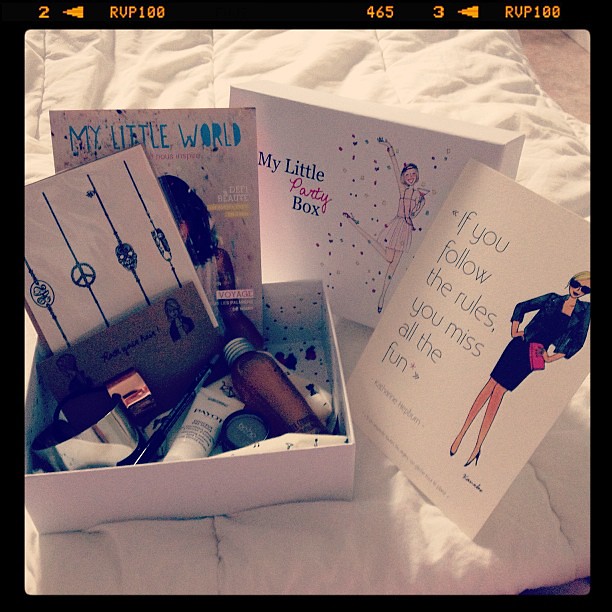This color photograph, distinctly tinted with a warm filter, showcases an inviting scene centered around a white cardboard box propped open on a white blanket, accompanied by a glimpse of carpet on the right edge. The box, boldly labeled "My Little Party Box," features a whimsical drawing of a girl sprinkling glitter while holding a drink. Surrounding the box is an array of thematic details that draw the viewer's attention. Positioned at the top of the image is a black border with notable orange text including "RVP100," and various numbers with directional arrows pointing towards them, adding a frame-like aesthetic to the picture.

On the lid of the box, there's an inspiring sign that reads, "If you follow the rules, you miss all the fun," next to a cartoon illustration of a tall, stylish white woman with short blonde hair, donned in black sunglasses, a sleek black dress, high heels, and a pink purse. The interior of the box reveals a mix of beauty products, including tubes of cream, makeup containers, and possibly body spray or perfume. The box is accented by white paper adorned with multicolored paint splashes, enhancing the festive atmosphere. This indoor photograph, bursting with light-hearted charm, captures a moment of playful elegance, likely representing someone's treasured makeup collection.